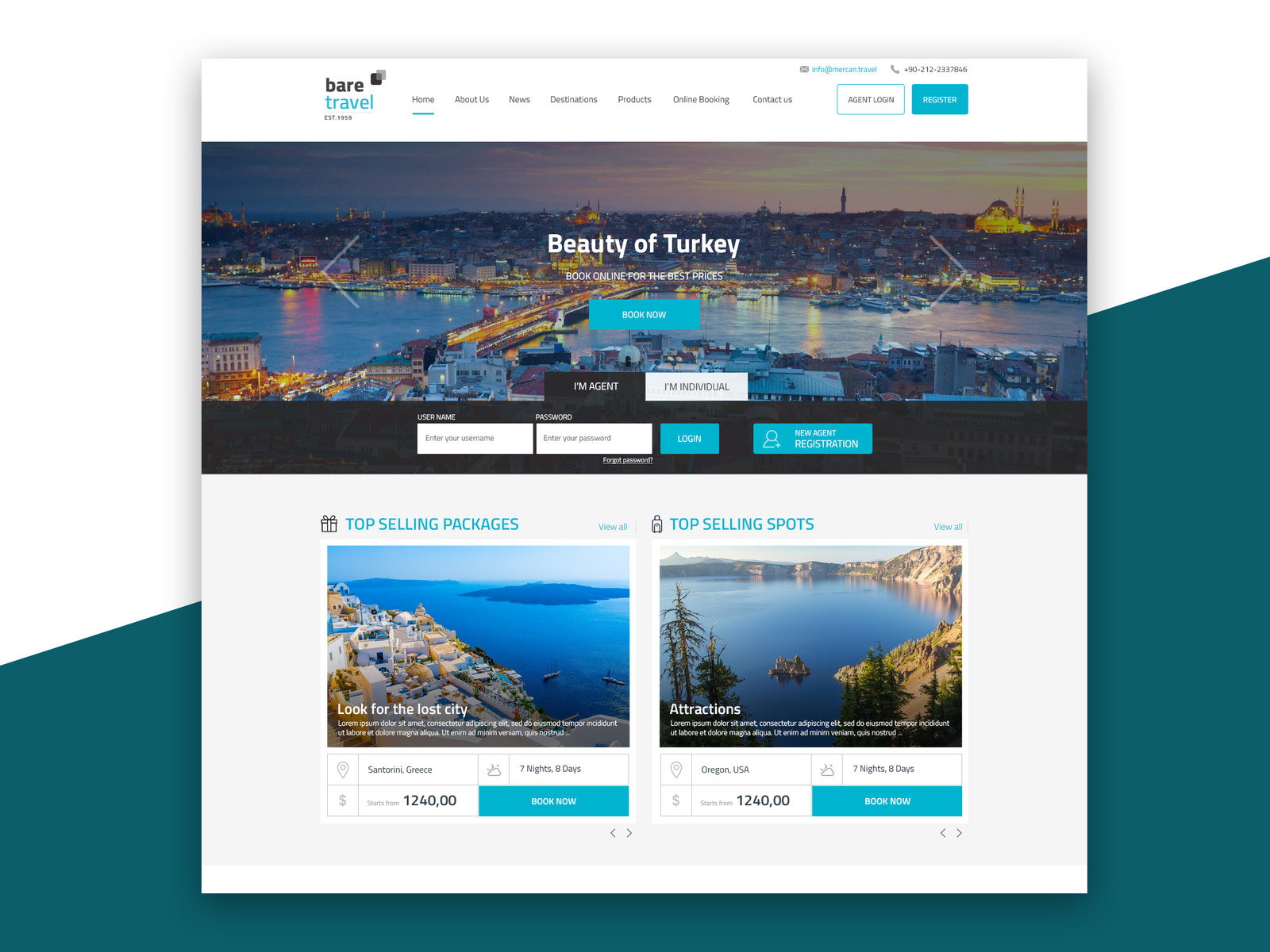In this well-crafted travel agency webpage, titled "Bear Travel," visitors are immediately greeted with a sense of history, noting that the agency was established in 1959. The header features an organized and intuitive navigation menu with drop-down options, including Home, About Us, News, Destinations, Products, Online Booking, and Contact Us. Essential contact details are prominently displayed in the top right corner, featuring the email address info@meccan.travel and the phone number +90-212-233-7846. 

Users can also find quick access links for agents to log in and register. Several captivating promotional highlights are showcased, such as "Beauty of Chorki," "Book Now," and a reminder to "Book Online for the Best Prices." The site emphasizes its top-selling sports and package deals, alongside a call to explore the intriguing "Lost City" attraction. The overall layout effectively combines practical information with enticing travel offers, making it easy for customers to plan and book their next adventure.